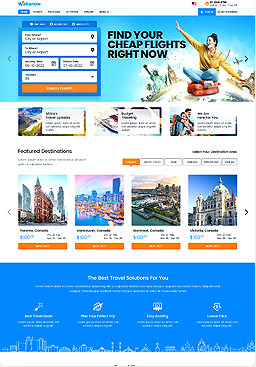The image shows a computer screen displaying a flight booking website. At the top center of the page, bold black capital letters read "FIND YOUR CHEAP FLIGHTS RIGHT NOW." Adjacent to these words, a young woman with dark hair styled in a bun is visible. She is wearing a long-sleeve gold sweatshirt and light blue jeans while sitting cross-legged on a red surface. Her outfit is completed with possible red socks and white shoes. She is posed with her arms mimicking the wings of an airplane—her right arm raised high and her left arm lowered.

The background of the screen features a blue sky with scattered white clouds. To the left of the woman, there is a blurred segment with a darker blue background that contains multiple white horizontal rectangles with black text, and an orange banner at the bottom.

In the center of the screen are seven icons, each representing a different city with accompanying descriptions and prices. At the bottom of the screen, a large blue banner with white text reads "The Best Travel Solutions for You." Everything except these words appears slightly blurry.